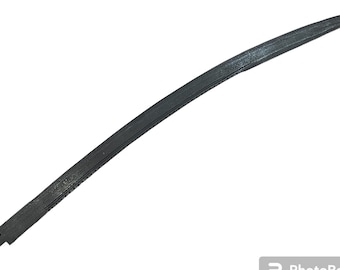The image displays a curved piece of black molding, potentially made of rubber, metal, or hard plastic, against a stark white backdrop. This molded piece arches from the bottom left to the upper right corner of the image, featuring fine striations across its surface. A shine creates brighter areas on the molding, particularly toward the bottom left and near the curve at the upper right. At the very bottom left, the molding forms a small V-shaped end, suggesting a layered structure. Additionally, a gray rectangle with indistinct white marks appears at the bottom right corner. The molding also exhibits a subtle kink in its otherwise sleek form, further enhancing its triangular appearance.